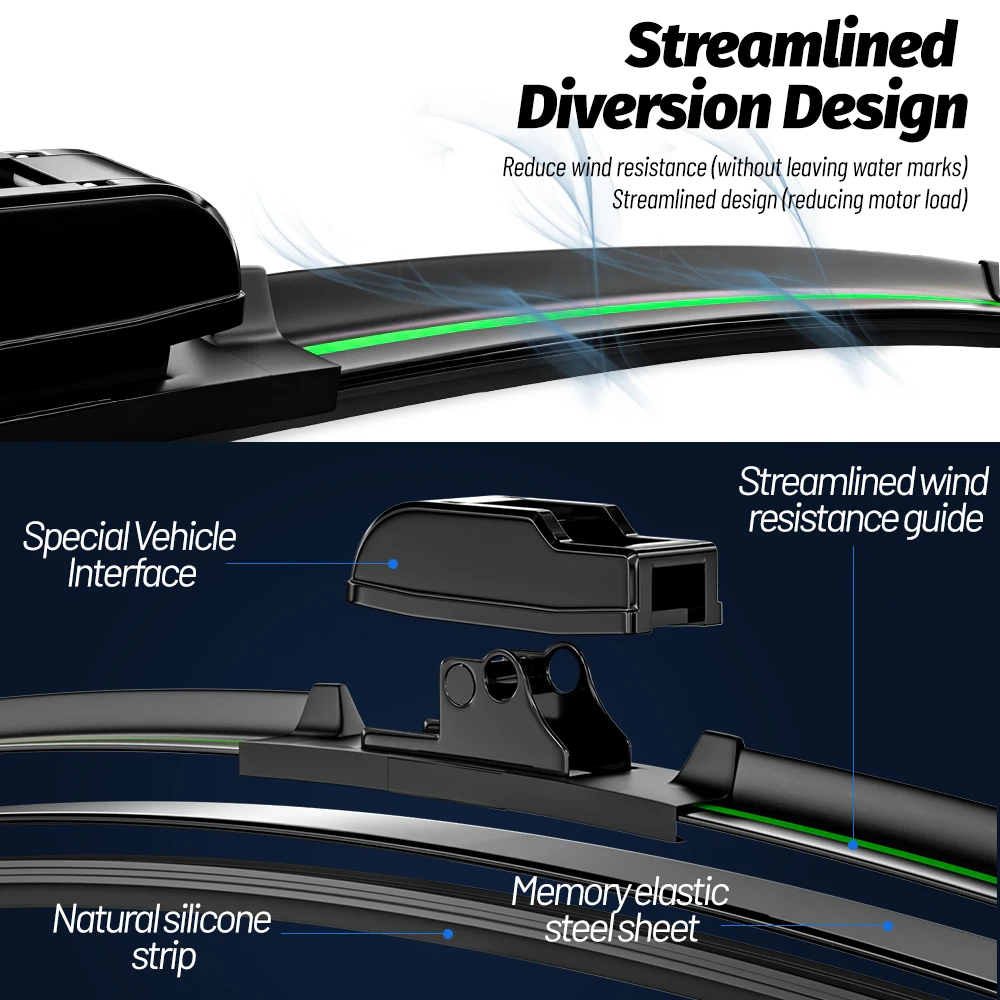This detailed and informative drawing showcases a set of windshield wipers designed for high performance. The image is divided into two main sections, each with descriptive text that highlights the innovative features of the wipers. 

The upper half of the image, set against a white background, emphasizes the blade itself. Prominently displayed in black capital letters are the words "Streamline Diversion Design," followed by the benefits of the design such as "Reduce wind resistance without leaving watermarks" and "Reducing motor load." The wiper blade is primarily gray, featuring a distinctive green band, and is depicted wiping away stylized blue streams representing water. 

The lower half of the image contrasts with a dark blue to black background, offering a closer look at the components of the windshield wiper. Key features include the "Special Vehicle Interface" and the "Streamlined Wind Resistance Guide." Focused illustrations show the detachable plastic cap and the wiper's frame with metal posts. The rubber strip of the wiper, which ensures a clean sweep, is labeled as a "Natural Silicone Strip," and the internal support is noted as a "Memory Elastic Steel Sheet." 

Altogether, this detailed depiction not only highlights the aerodynamic and functional aspects of the wiper blades but also underscores the advanced materials and engineering that reduce motor load while ensuring a streak-free performance.